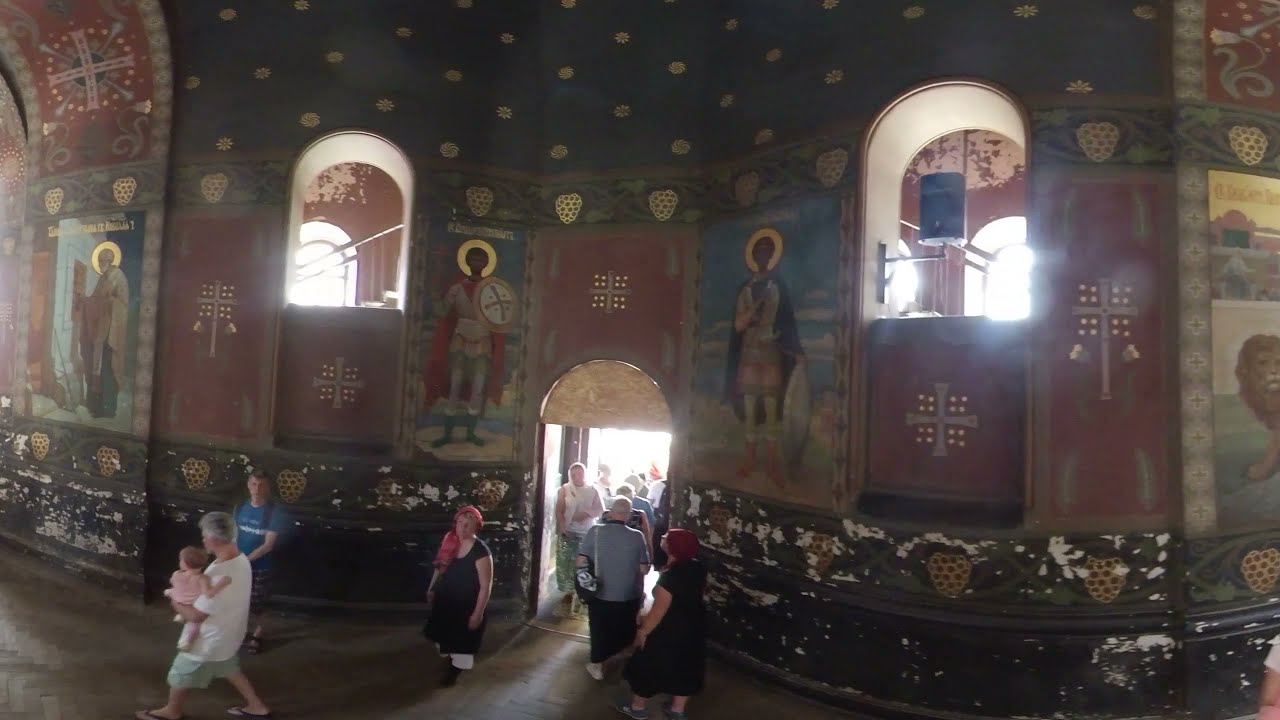The photograph depicts the interior of an old church adorned with intricate art and religious iconography. The walls are richly decorated with ornate murals and mosaics, featuring Christian figures with gold halos, indicating their sanctity. The art exudes a Byzantine or pre-Byzantine aesthetic, with dominant hues of blue, burgundy, and gold. The lower portions of the walls show signs of age, with dark, brown, and gray paint peeling away.

In the center of the image is an arched doorway through which people are entering and exiting. Among them, a man can be seen carrying a baby dressed in pink, alongside families and individuals of various ages. The scene captures the dynamic flow of visitors, bathed in bright light from outside, contrasting the dark interior. High above, two arched windows let in additional light, and the upper sections of the walls are adorned with decorative motifs, completing the sacred and historical atmosphere of the church.